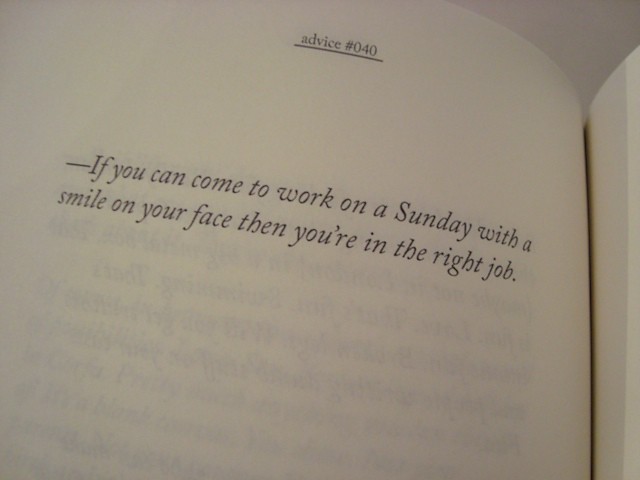The photograph captures an open book, positioned nearly halfway through. The page, which is an off-white color and appears thin enough for the black text from the opposite side to faintly show through, features a small, underlined heading at the top that reads "advice no. 040." Below the heading, a dash precedes the italicized text: "If you can come to work on a Sunday with a smile on your face, then you're in the right job." There is a visible shadow in the crease of the book, and the background in the upper right corner is a light gray. No citation accompanies the quote, and the rest of the page remains blank, contributing to a minimalist aesthetic.